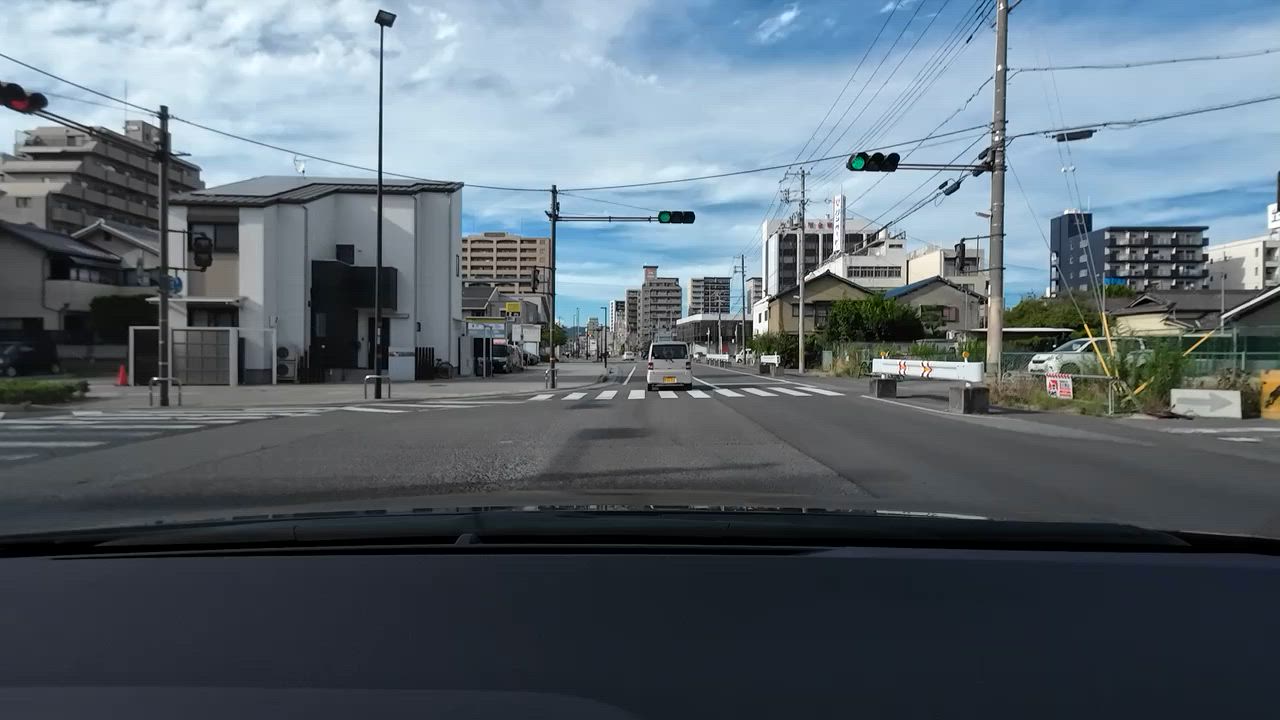From the driver's perspective, the scene captures the essence of navigating a bustling city street. Through the windshield and over the dashboard, you see a significant main street, bustling with urban life yet void of immediate traffic. Streetlights extend horizontally from both sides, arching over a wide crosswalk. In the distance, a skyline dotted with towering buildings hints at a mix of residential apartments and commercial businesses, looming on both the left and right. To the right, a white guardrail traces the edge of the road, punctuated by several telephone poles standing sentinel. The sky above is an expanse of vibrant blue, accented with scattered clouds, providing a serene backdrop to the urban landscape. The traffic lights ahead shine green, guiding the way forward.